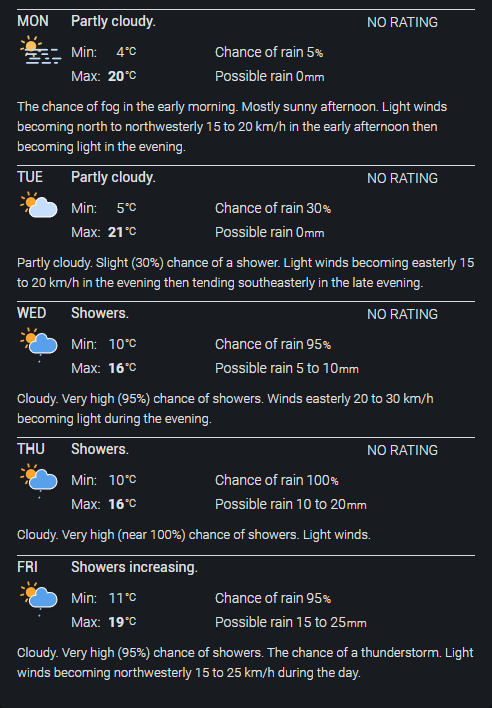The image is a neatly organized, black-background screenshot displaying a five-day weather forecast in Celsius. The forecast is divided into five sections, each separated by thin white lines, with white font making the details easily readable. At the top left corner of each section, the first three letters of the day are indicated.

Each day's forecast includes a weather icon that visually represents the day's predicted weather conditions. Immediately to the right of the day, detailed descriptions such as "partly cloudy" or "showers increasing" are provided. Below each description, the minimum and maximum temperatures for the day are listed, with the maximum temperature bolded for emphasis. 

To the far right, the forecast gives the percentage chance of rain, along with a detailed breakdown of the expected rainfall in millimeters. There is also an additional blurb at the bottom of each section, providing more specific information about the day's weather patterns. 

For example, the forecast for Monday reads as follows: 

- Icon depicting partly cloudy conditions.
- Description: Partly cloudy.
- Temperatures: Minimum of 4°C, Maximum of 20°C (bolded).
- Rain: 5% chance with 0 millimeters expected.
- Additional details include: "Chance of fog in the early morning. Mostly sunny in the afternoon. Light winds becoming north to northwesterly at 15 to 20 kilometers per hour in the early afternoon, then becoming light again in the evening."